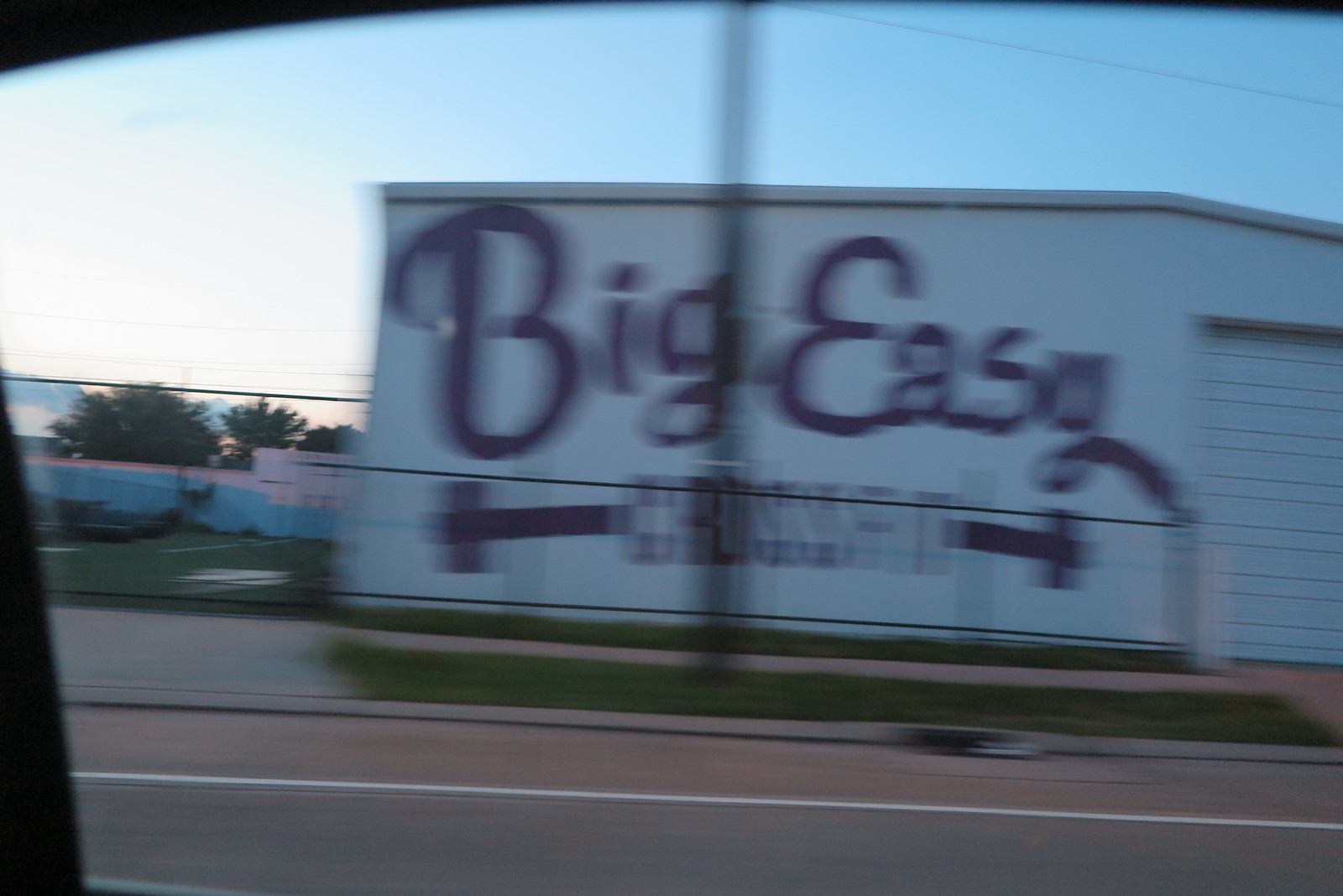A photograph captured from a swiftly moving vehicle showcases the side of a predominantly white warehouse-like building. Prominently displayed on the building is a sign for "Big Easy," although the text beneath it is indiscernible due to blurriness. To the right, the structure features a typical warehouse garage door. While the vehicle itself is mostly out of the frame, the window's edge is visible, emphasizing the motion through the surrounding blur. The clean street in front of the building includes a drain and a light pole. Additionally, there is a sidewalk with a patch of well-kept grass adjacent to the street.